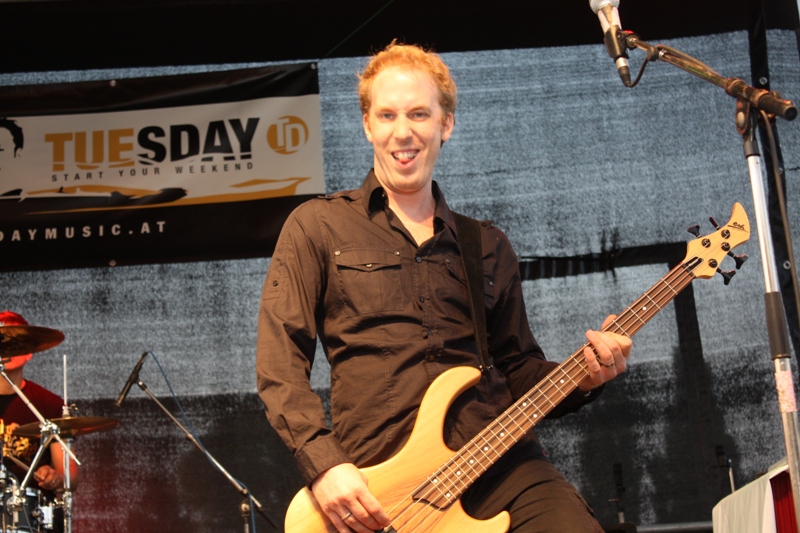In the center of the stage, a white male with reddish-brown hair and a slightly balding head is energetically playing a large, wooden-colored bass guitar. He is dressed in a black button-up shirt, with the top button undone, and the shirt features pockets on the front. He has his left fingers on the strings, while his right hand is picking the strings. His knee is propped up on something, adding to his dynamic pose. He has a ring on his right hand and another on his left, visible as he plays. His tongue peeks out from beneath his teeth as he smiles broadly, glancing at the camera. 

To his right, a microphone on a stand is visible in the foreground. Behind him, to the left, there is a drummer in a brown shirt playing on a mic'd up drum set with visible cymbals. The drummer’s face is partially obscured. 

The backdrop features a large black curtain with a gray mottled pattern and a black rectangle towards the bottom. A banner hangs on the curtain, reading "Tuesday, start your weekends," although it's somewhat hard to read due to its distance. The banner has a white stripe bordered by black stripes, with abstract elements, including partial faces and lettering in black and brown.

Overall, the stage is set for an engaging musical performance with a joyful and lively atmosphere.